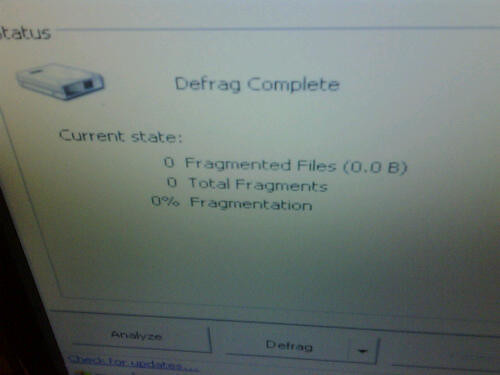A photograph captures a computer screen displaying an outdated defragmentation status pop-up. The white background features black text in the upper left corner that reads "Status: Defrag Complete." Below that, the current state is detailed with "0 fragmented files," "0.0 bytes," "0 total fragments," and "0% fragmentation." On the left-hand side is an icon resembling a disk or hard drive. Under these details, there are two buttons: "Analyze" on the left and "Defrag" with a dropdown arrow on the right. Below these buttons, a blue hyperlink allows the user to "Check for Updates." The close-up angle of the photograph highlights the obsolete style of the text, reminiscent of an older machine system.